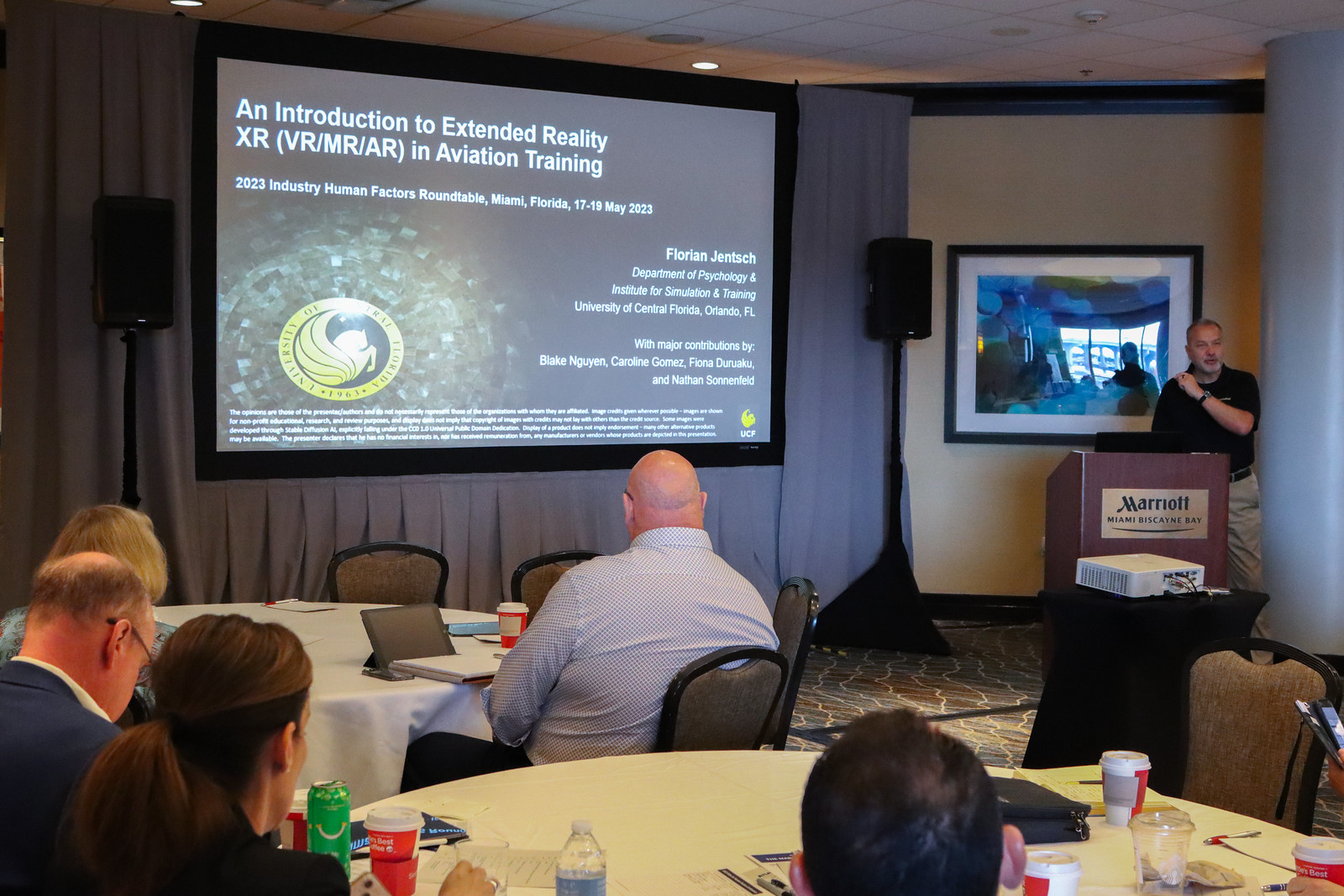This photograph depicts a dynamic scene at a conference panel held in a Marriott hotel conference center, specifically the Marriott Miami Biscayne Bay. The room features round tables covered in white tablecloths, scattered with items such as papers, coffee cups, pens, glasses of water, and an iPad held by a bald attendee. The participants, numbering around four to five in the visible area, are attentively seated, engrossed in the ongoing presentation.

A man, presumably in his 50s, with grayish hair and a matching beard, stands behind the podium to the right side of the image. He is dressed in a short-sleeved black polo shirt and light brown khakis, secured with a belt. The podium prominently displays the "Marriott Miami Biscayne Bay" label. Mounted on poles, two speakers flank each side of a large projector screen on the left side of the image.

Displayed on the projector screen is a title slide for the presentation, which reads: "An Introduction to Extended Reality (XR) (VR, MR, AR) in Aviation Training." This slide further specifies that it is part of the "2023 Industry Human Factors Roundtable, Miami, Florida, 17-19 May 2023." The presenter's name, "Florian Jentsch, Ph.D.," is listed alongside his affiliations with the Department of Psychology and the Institute for Simulation and Training at the University of Central Florida, Orlando, Florida. Additional contributions to the presentation are credited to Blake Nguyen, Caroline Gomez, Fiona Do, and Nathan Simonfield. A painting behind the speaker reflects the scene in the opposite direction, adding depth to the setting.